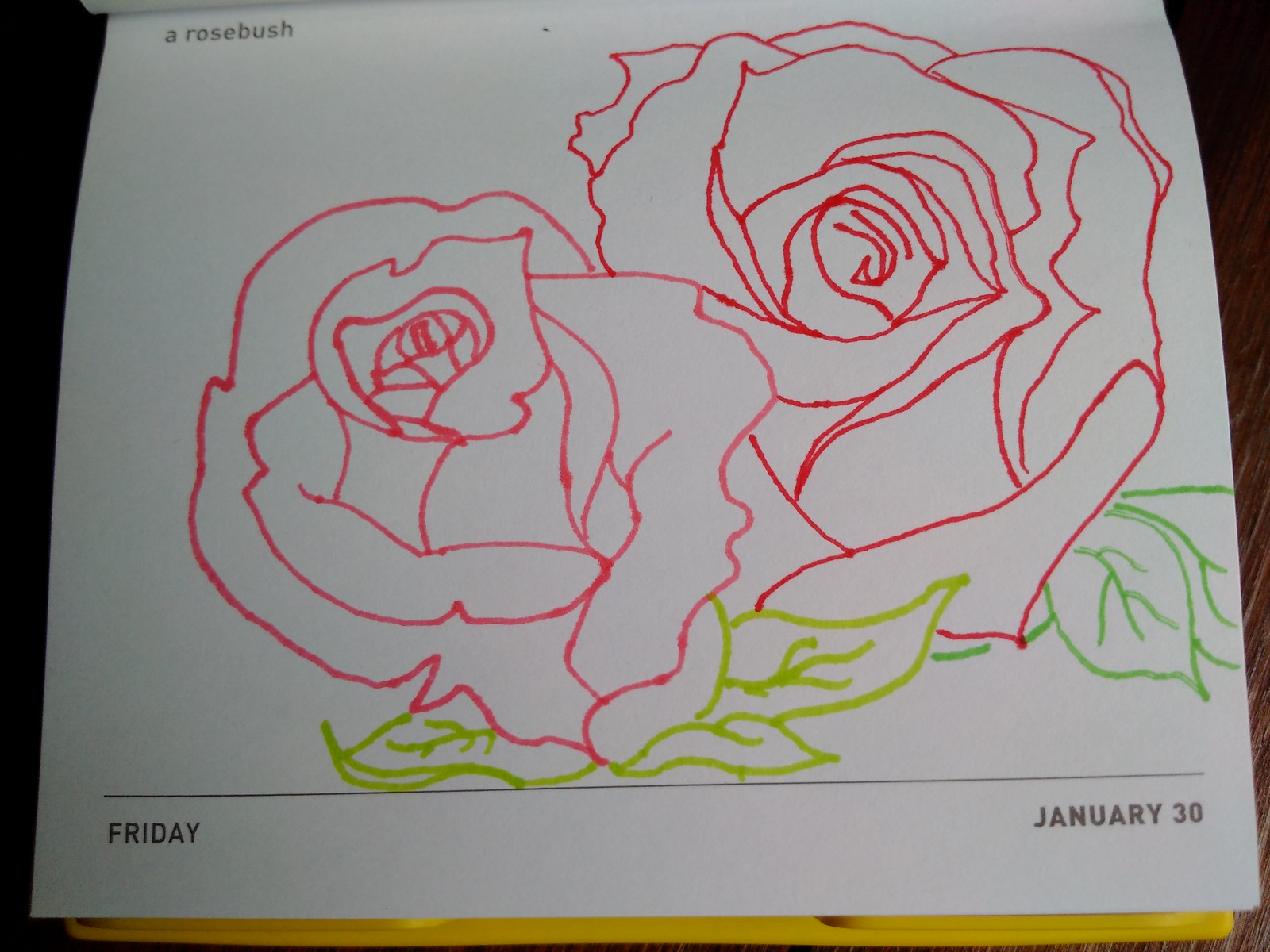The image depicts a slightly wider-than-tall photograph featuring a desktop calendar against a black background. The off-white page at the forefront resembles a daily flip calendar, with a yellow backing visible at the bottom. At the top left of the page, "a rosebush" is printed in small, subtle gray letters. The paper showcases a simplistic sketch of two fully bloomed roses: one on the left is drawn in light pink, and another on the right is sketched in a darker red. The roses, facing somewhat towards the viewer, are adorned with corresponding leaves—light green on the left and darker green on the right. Below the sketches, a thin black line runs horizontally across the page. In the bottom corners, "Friday" is printed in black uppercase letters on the left, and "January 30th" in the same style on the right. The drawing is akin to a coloring page, perhaps intended for a young child's activity booklet, awaiting colorful embellishments to be added.